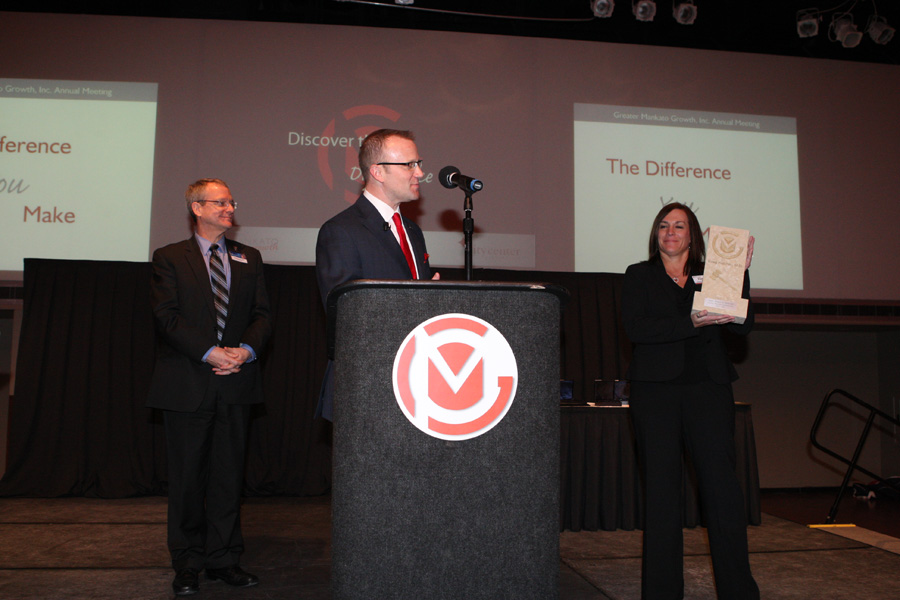The image shows a conference presentation featuring three individuals standing in an auditorium. At the center, a gentleman in a suit stands at a dark gray podium with a circular logo combining the letters "C" and "M" in red and white. He is gazing to the right. To his left, another man in a dark suit with a striped tie stands attentively. To his right, a Caucasian woman in a dark suit holds a large rectangular beige object, possibly an award. Behind them, a projector screen displays a presentation with a dark red background featuring the words "Discover the Difference" in black and red. White squares on either side of the screen contain the phrase "the difference you make," where "difference" and "make" are in red and "you" is in gray. The central figure partially obstructs the view of the full text on the screen.